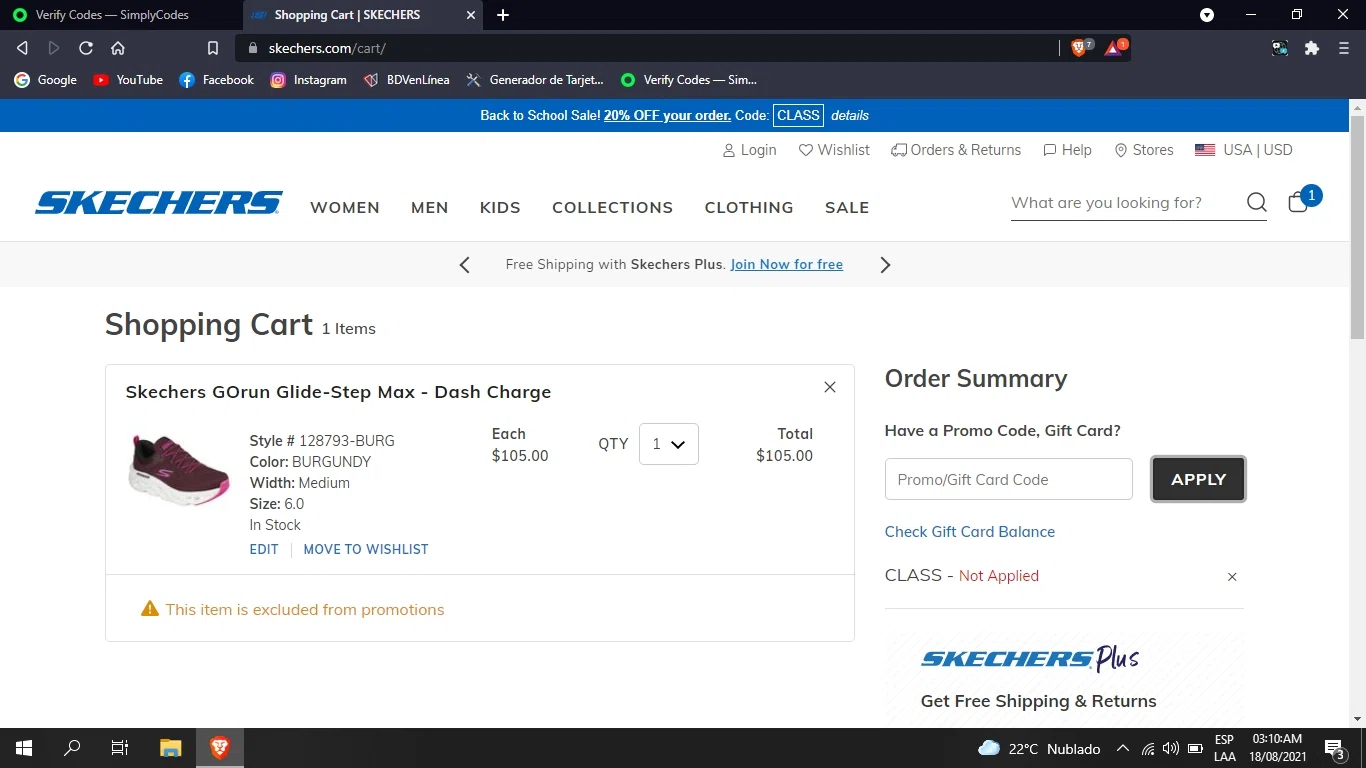This is a detailed screenshot of the Skechers website. At the top, the brand name "SKECHERS" is prominently displayed in all capital blue letters. Adjacent to it, in black text, are navigation links labeled "Women," "Men," "Kids," "Collections," "Clothing," and "Sale." Below this menu, the site indicates "Shopping Cart, One Item."

The central area features a striking image of a burgundy-colored shoe, identified as the "Skechers Go Run Glide-Step Max Dash Charge," priced at $105. Directly beneath the shoe's description, there is a quantity box showing the number 1. To the right of the shoe description, there is a heart icon accompanied by the word "Wish List."

Additional icons are displayed along the top interface:
- A small truck next to "Order and Returns."
- A chat bubble next to "Help."
- A location pin next to "Stores."
- A small American flag followed by "USA, USD."

There is a concise visual of a shopping cart with a blue circle highlighting the number 1, indicating an item in the cart. A search bar features the text "What Are You Looking For?" adjacent to a magnifying glass icon. Finally, a black rectangle with the white word "Apply" is prominently visible, likely part of a call-to-action or promotional section.